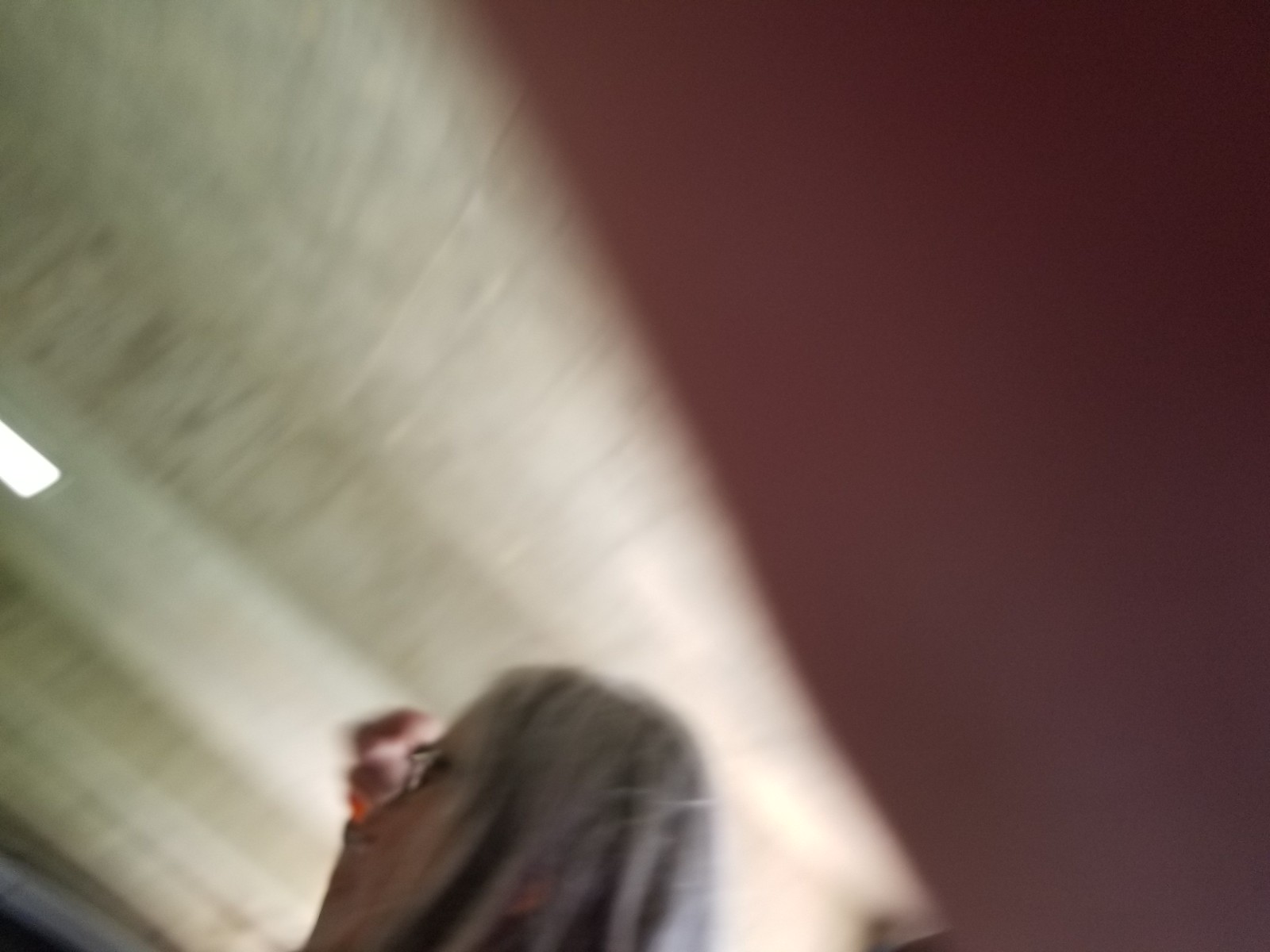A slightly out-of-focus and covertly taken image shows an individual, most likely a woman with long, straight grey hair and black glasses, positioned at the lower left of the frame. She appears to be a white lady, possibly with darker hair underneath the grey, and her hand is raised in the air, maybe gesturing or in motion. The photograph is taken from a low angle, suggesting it was stealthily captured from the photographer's lap. The background features a white wall with a bright rectangular light source along the left side and darker, possibly maroon or brown, sections to the right. The image's composition is slanted slightly counterclockwise, adding to its covert and hurried nature, consistent with the impression of the photographer trying to be inconspicuous, perhaps due to the belief that the woman might be yelling or reacting strongly. The setting could possibly be inside an airplane, given the visible ceiling and the ambient lighting, though this is difficult to confirm.